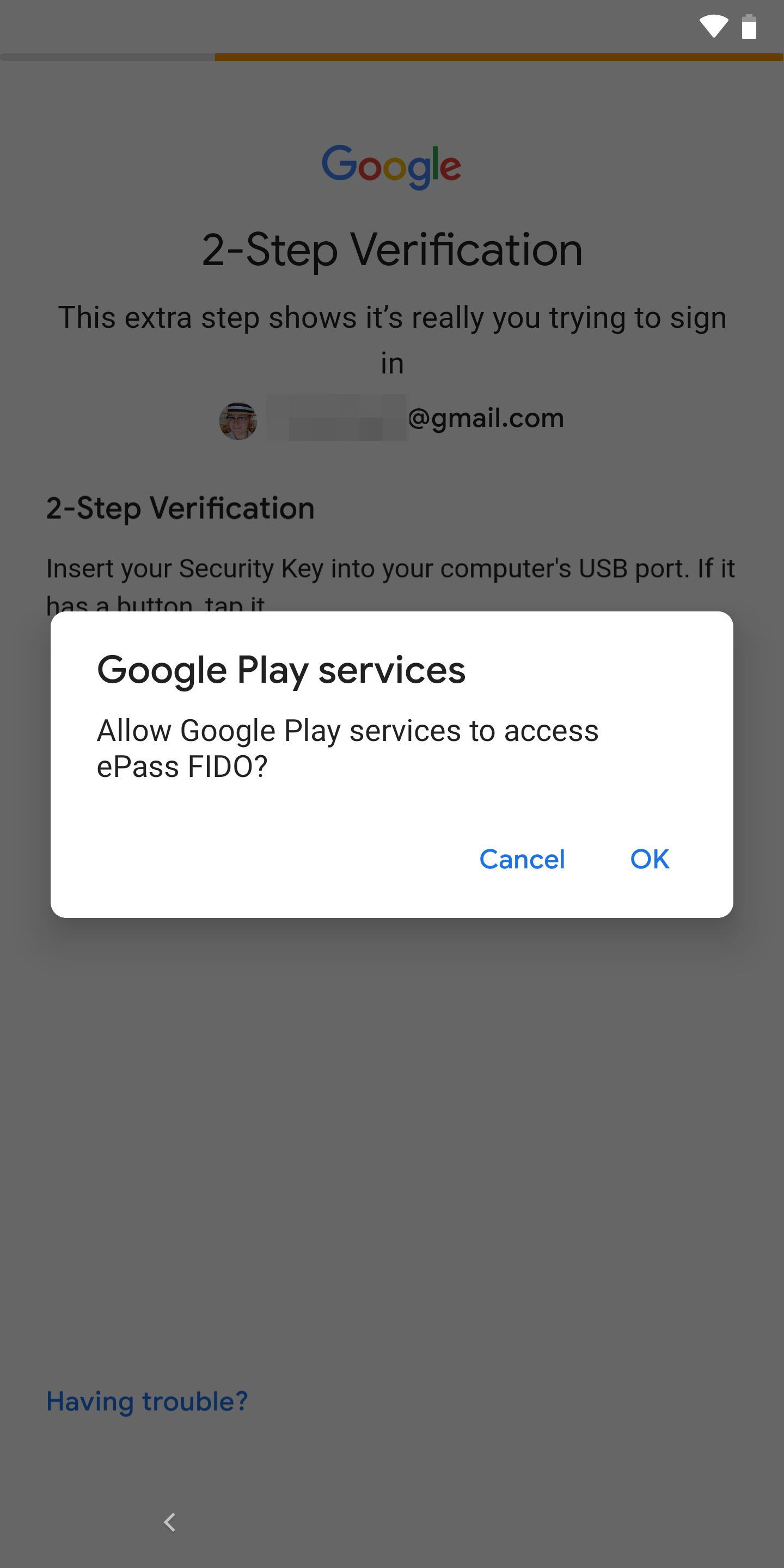The image showcases a blurred-out background, primarily in grayscale, overlaid by a Google security prompt. At the top, the Google logo is visible next to a bolded "Two-step verification" title. Beneath this title, a non-bolded subtitle reads "This extra step shows it's really you trying to sign in." The display includes a profile picture and a partially blurred-out email address, revealing only the "@gmail.com" domain. Below, the instructions for two-step verification suggest inserting a security key into the computer's USB port, though the full text is obscured by a pop-up.

The prominent pop-up box has a white background with bolded text reading "Google Play services." The subsequent text, in a lighter gray font, asks, "Allow Google Play services to access e-pass FIDO?" with options "Cancel" in blue on the right-hand side and "OK" in the bottom-right corner.

Returning to the grayed-out background, near the bottom-left corner, a hyperlink reads "Having trouble?" with a question mark. The very bottom of the screen shows a small white back arrow.